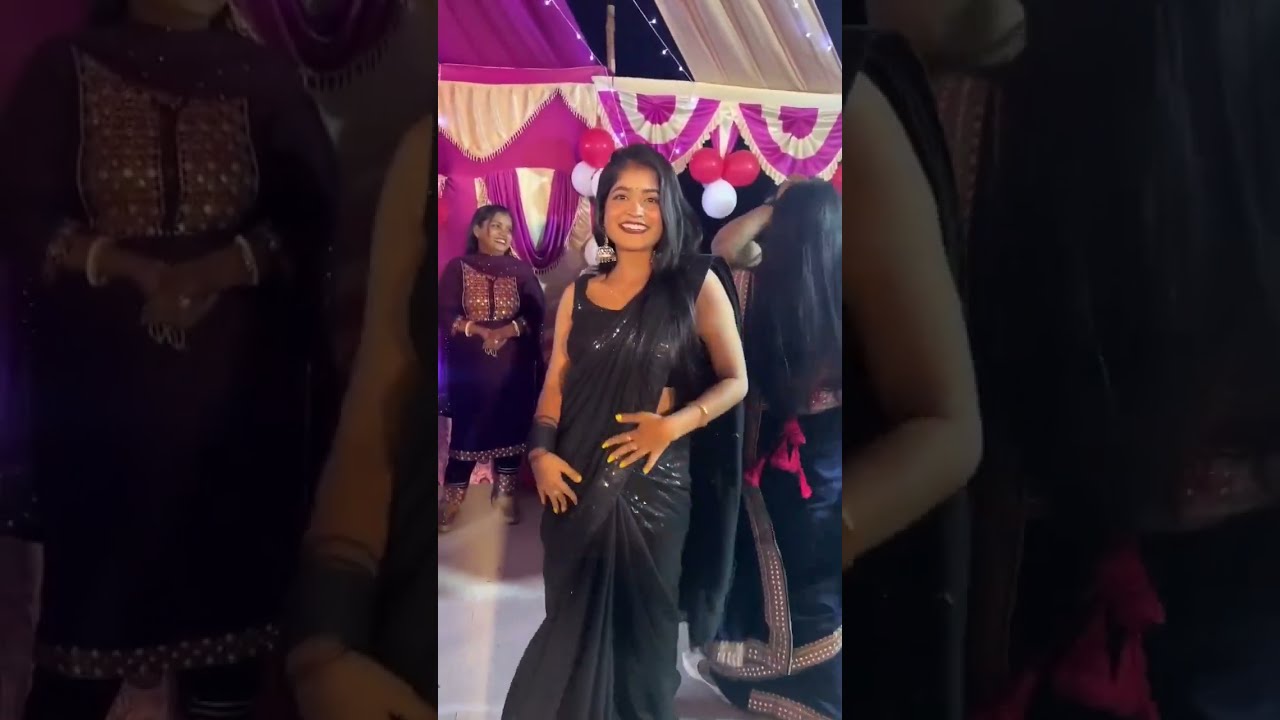The image is a vertical cell phone style picture depicting a woman at a party, set against a creatively zoomed-in and faded background of the same scene. The main woman, possibly of Indian descent, stands about 5 feet from the camera, smiling warmly. She is adorned in a formal, sleeveless, dark-colored dress that fully covers her body and slightly flares out at the skirt. Her dress appears to be accentuated with sparkly elements, resembling a black sari dress with a sports cropped top and sash over her left shoulder. She accessorizes with a long dangly earring on her right side, black bangles on her right wrist, a gold bangle on her left wrist, and yellow fingernail polish.

Her long, straight black hair cascades over her shoulders, some strands resting in front while the rest is tucked behind. The party environment in the background features a pink and white tent with banners and two other women—one with her back turned and another facing forward but looking away. The photograph also exhibits a unique framing effect, using enlarged and darkened versions of the background image on the left and right sides, highlighting the festive atmosphere.